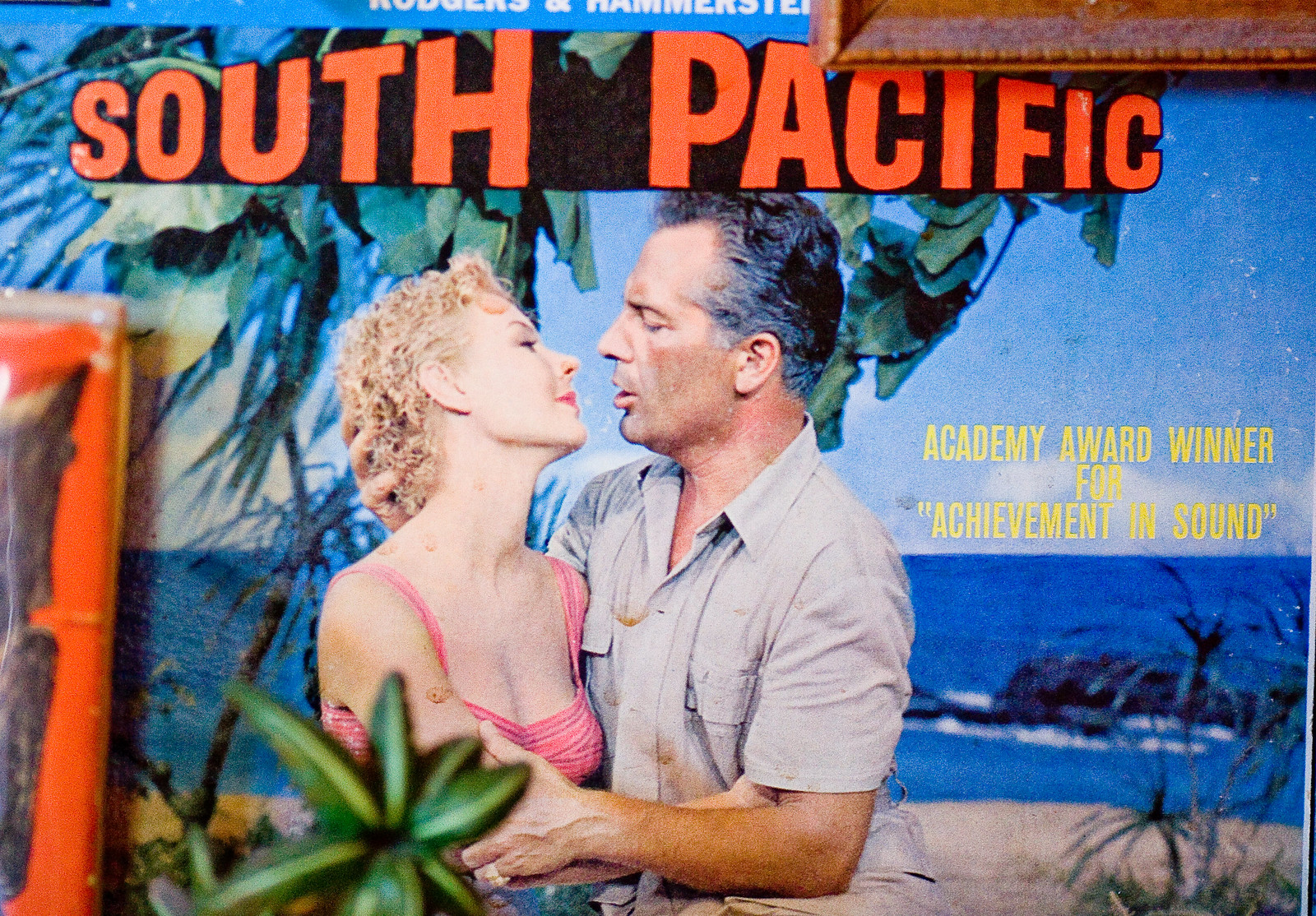In this vibrant, colorful poster for the musical "South Pacific," a man and a woman are captured in an intimate embrace, their faces mere inches apart as if they are about to kiss. The woman, with her head slightly tilted back, flaunts short, curly, dirty blonde hair, and is dressed in a spaghetti strap pink top. She radiates happiness with a smile, while the man, an older figure with hints of gray in his black hair, wears a button-up khaki shirt and holds her closely, his expression serious. The backdrop features a meticulously staged, tropical island scene showcasing a beach with palm trees, ocean waves crashing against rocks, and sandy shores. The text "South Pacific" is prominently displayed in orange above their heads, while to their right in yellow, it reads "Academy Award Winner for Achievement in Sound." This advertisement fills the entire frame, invoking a nostalgic, beach-themed ambiance reminiscent of a classic movie or theatrical production from decades past.